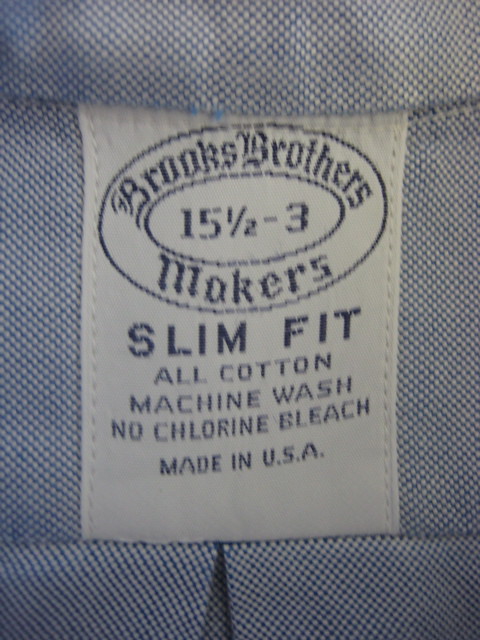This image features a close-up photograph of a white rectangular clothing tag sewn into a garment with tiny black and white checkered fabric in a criss-cross pattern. The fabric's intricate design is accentuated by the alternating tiny black and white threads. At the center of the image, the tag prominently displays "Brooks Brothers Makers" in a dark blue circular emblem. Inside this emblem, the size "15.5-3" is featured. Below this, the bold text "Slim Fit" stands out, followed by the details "All Cotton," "Machine Wash," "No Chlorine Bleach," and "Made in USA." The tag is meticulously stitched onto the fabric and gives a clear sense that this is likely part of a shirt due to the design and placement of the tag.